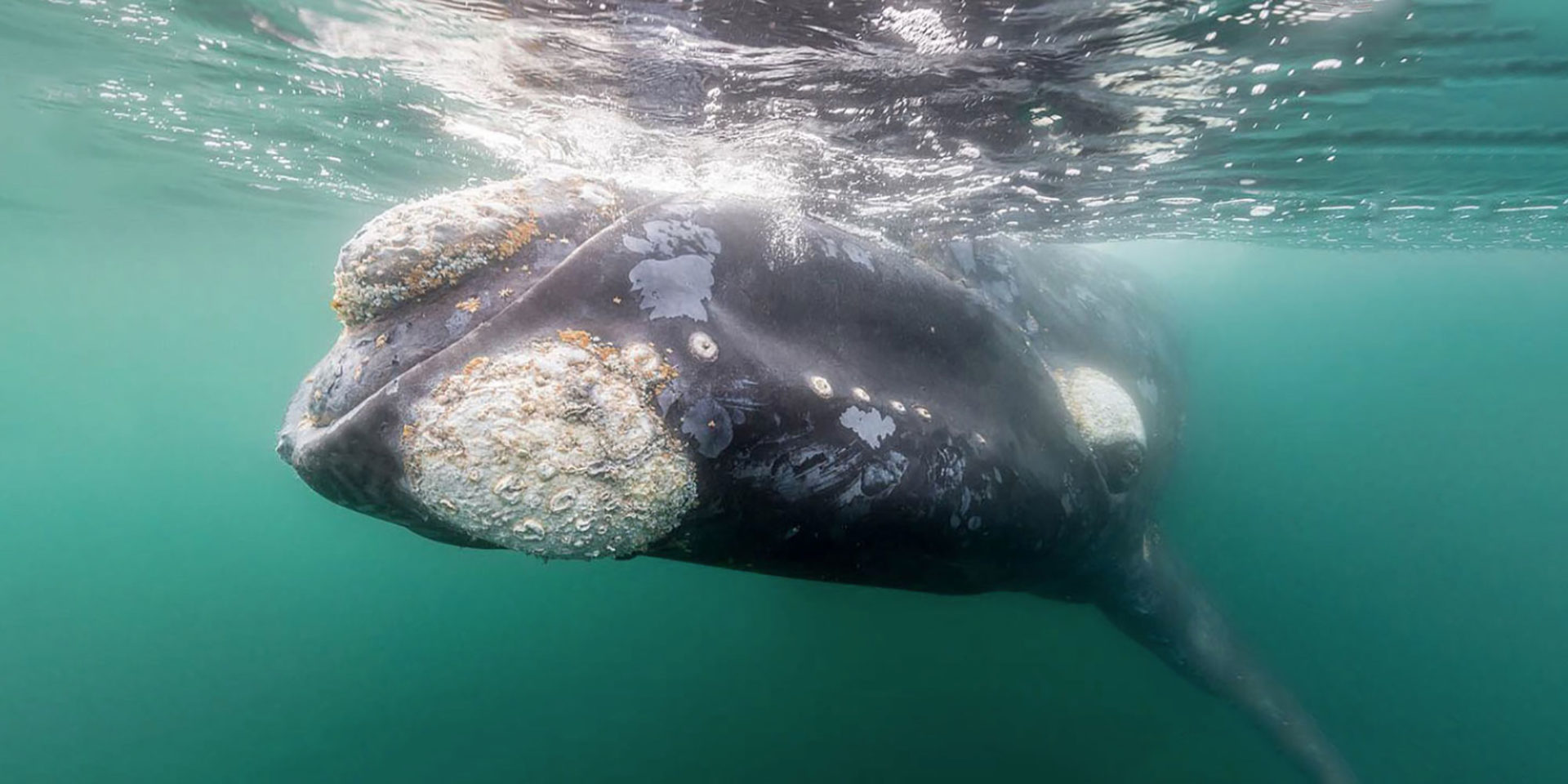This underwater color photograph captures the head-on approach of an old humpback whale swimming in clear, teal-green water near the surface. The whale, prominently positioned in the center, has a dark gray body marred with lighter gray scars from previous wounds. Its face is heavily encrusted with white and brown barnacles, particularly around its nose and near its chin, alongside patches of algae. The large, bulbous eye appears curious and might even be closed, partially obscured by barnacles. A single fin is visible on the lower right side of the image, pointing downward. The water above displays ripples and light refraction, indicating the proximity to the surface, while the cloudy and hazy backdrop adds depth to the photograph.